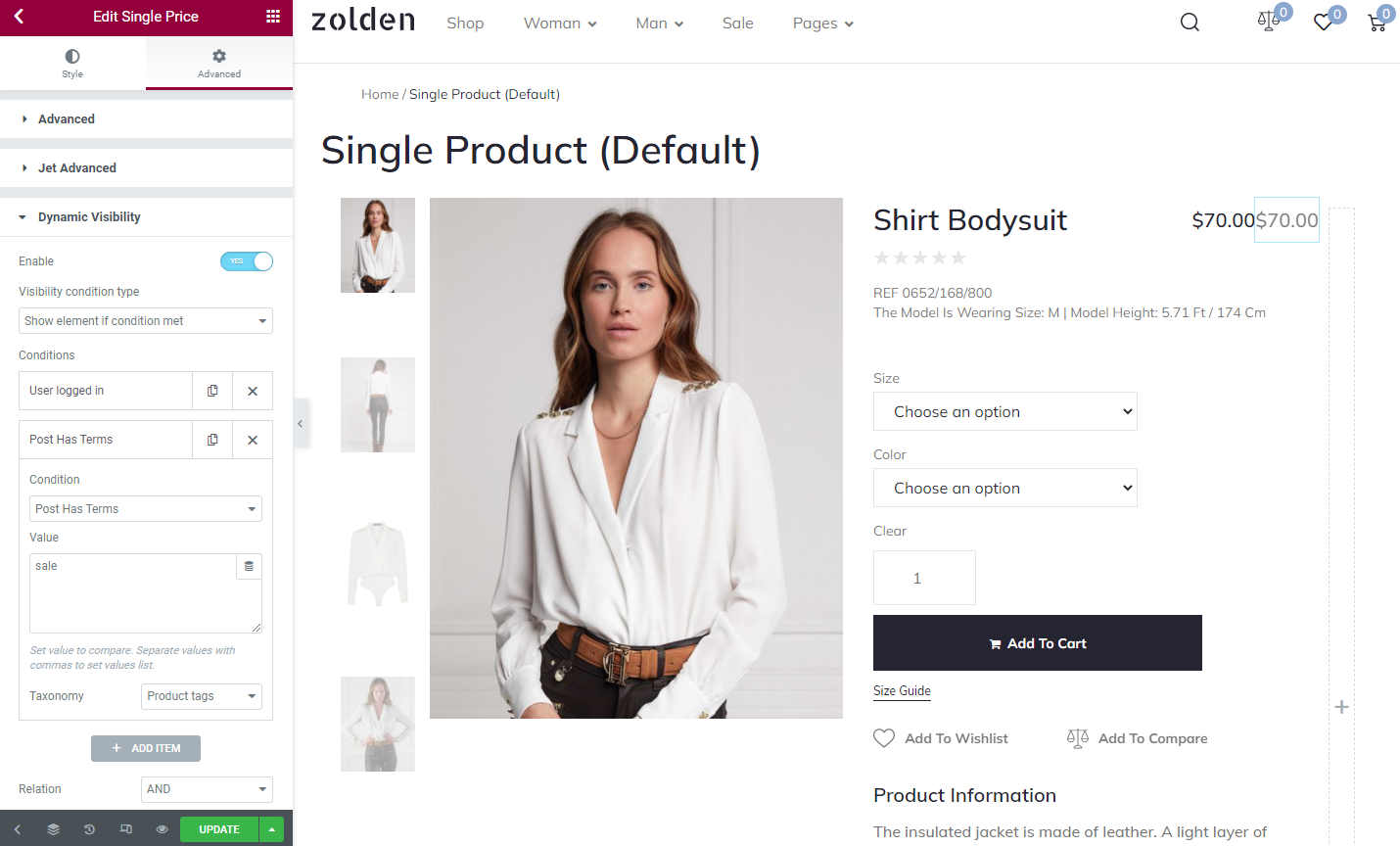The image comprises two screenshots side by side. The screenshot on the left depicts a smartphone app interface, where the settings for a product listing are visible. It includes options such as "Edit Single Price," "Advanced," "Jet Advanced," and "Dynamic Visibility," indicating functionalities for modifying the product details.

The screenshot on the right displays the website interface of Zolden (spelled Z-O-L-D-E-N). Centered prominently on this page is a fashion model dressed in a white, long-sleeved shirt, paired with a brown belt and blue jeans. Above the model, the text "Single Product (Default)" is prominently displayed. Below this, there is a product description stating "Shirt Bodysuit, $70."

This detailed depiction suggests that the left screenshot shows the mobile app settings used for adjusting the listing seen on the Zolden website, ensuring dynamic and advanced control over the product's presentation and pricing.